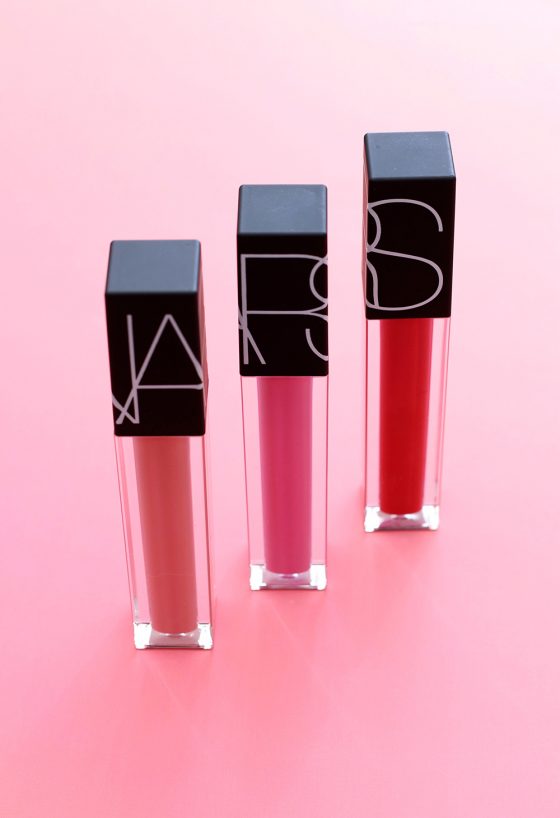This photograph features a product display set against a stylized pink background that fades from light at the top to darker at the bottom middle. The image showcases three tall, rectangular containers, which appear to be nail polish or possibly lipstick, arranged at an angle. Each container is square-shaped with a black lid that features partial lettering, suggesting the letters 'N', 'A', 'R', and 'S'. The bottom portions of these containers are made of clear plastic, revealing the vibrant colors within: one is peachy pink, another is a bold pink, and the third is a rich red. The branding on the black lids seems to spell out "NARS," though it is fragmented and not entirely clear.